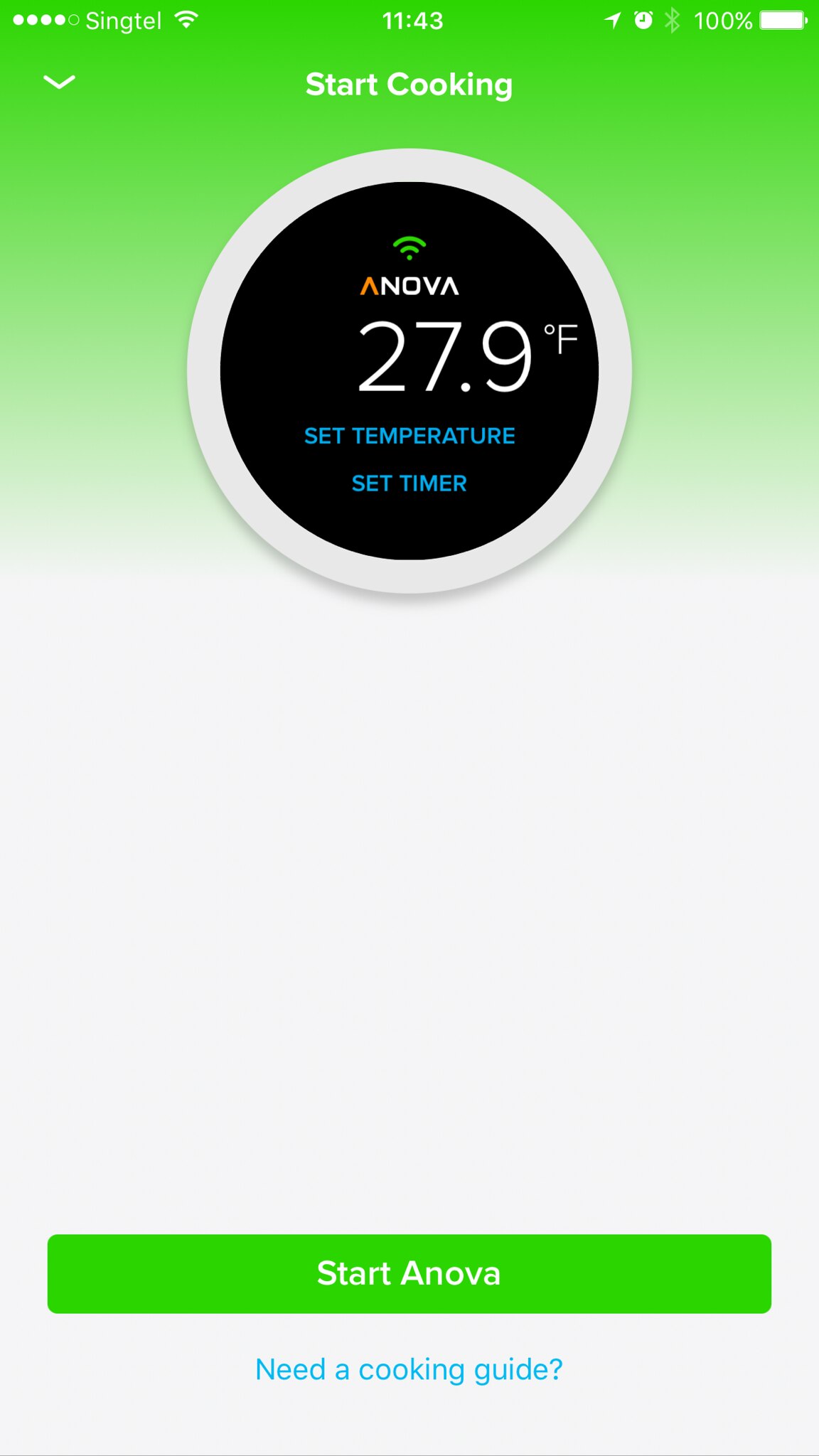The image appears to be a screenshot of a cooking app interface on a smartphone. The background starts with a green gradient at the top, transitioning into white as it moves downward. 

At the top portion of the screen, there's a section with icons: several white circles and a green circle accompanied by some text that is illegible. There is also a sound bar icon beside these elements. 

In the center of the interface, in the green part, it displays the time as "11:43 AM," next to which is a white circle bearing an unreadable icon and some symbol in light green, followed by the text "100%". Adjacent to this, there is a white rectangle. Below this section, a button labeled "Start Cooking" is prominently displayed. 

Further down, closer to the bottom, there is another larger green rectangle containing the text "ANOVA" with "A" in orange and the remaining letters in white. Underneath, in smaller blue text, it reads "Need a cooking guide?"

At the very bottom of the interface is a black-filled white circle featuring three curved green lines, and to its right, the label "ANOVA" appears again, formatted similarly with the "A" in orange and the subsequent letters in white. Beneath this, there are instructions in blue text reading "Set Temperature" and "Set Timer," along with the notation "27.9°F" in white.